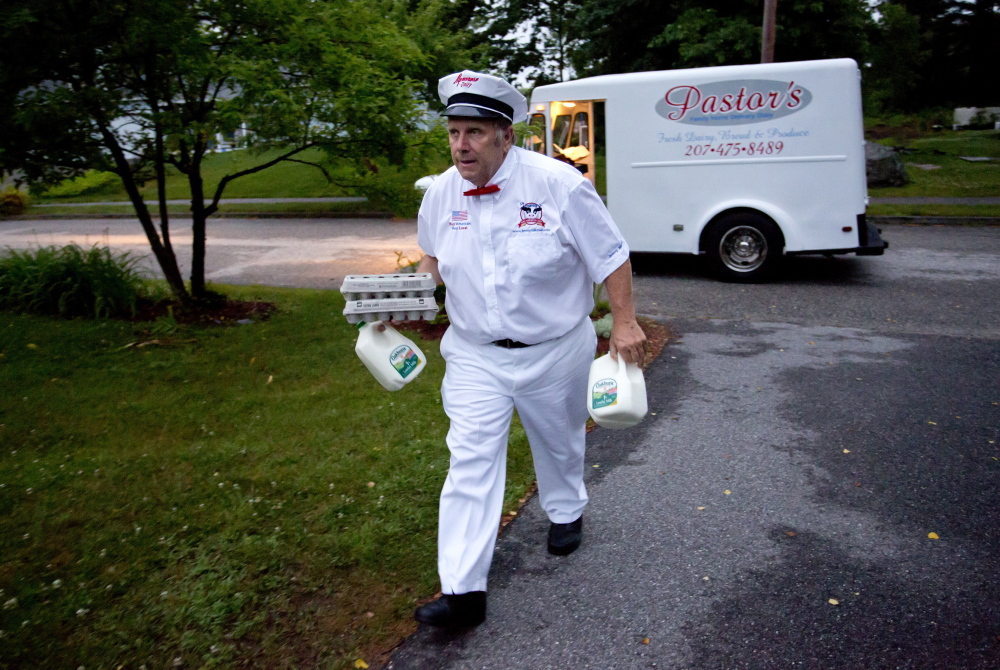This vintage image captures a scene of a traditional milkman making a delivery in a typical American suburb. The setting appears to be at dusk or dawn, suggested by the low light and the wet pavement, possibly from recent rain. The milkman, a slightly overweight Caucasian gentleman in his late 60s with gray hair and no facial hair, is walking up the driveway of a home. He is dressed in an all-white outfit comprising a white hat with blue and black rims, a white button-down shirt with sleeves rolled to the elbows, white pants, black shoes, and a distinctive red bow tie. On his uniform, he sports an emblem above his pocket and an American flag on the left side. In his right hand, he carries two cartons of eggs and a gallon of milk balanced on his wrist, while in his left hand, he holds another gallon of milk. Behind him, parked on the road, is a white truck labeled "Pastors" along with a telephone number 207-475-8489, written in red and blue text. The backdrop of the image features suburban elements such as green lawns, trees, and houses. The milkman, embodying a bygone era, diligently walks up the driveway against this quaint and nostalgic setting.